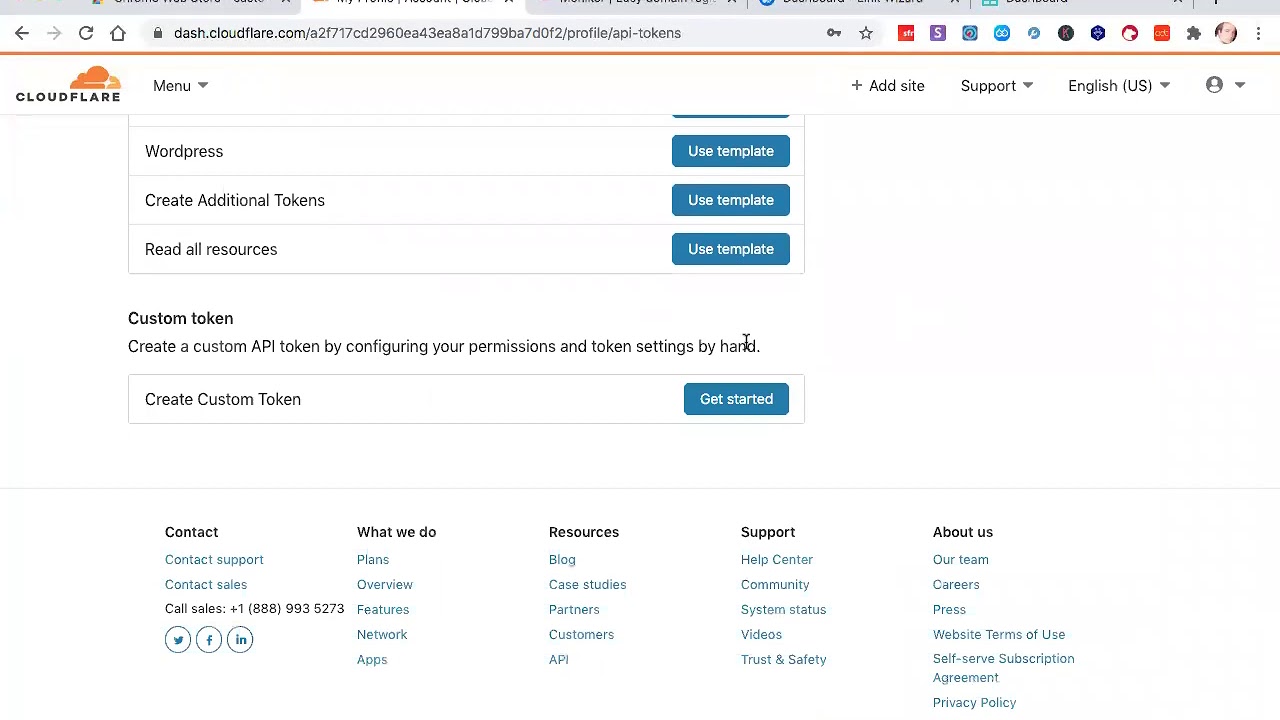The image displays a screenshot of a user navigating the Cloudflare dashboard via a web browser, evidenced by the URL "dash.cloudflare.com" visible in the browser's tab. The Cloudflare logo, designed as an orange cloud, is prominently featured on the page. 

The user interface includes a variety of navigation options and functional elements geared towards web developers and site administrators. Notably, there is a section dedicated to WordPress, with an adjacent blue box labeled "Use Templates" for quickly deploying predefined setups. Similar "Use Templates" options appear next to menu items such as "Create Additional Tokens" and "Create All Sources," suggesting an emphasis on streamlined workflows for common tasks. 

Further down, the dashboard presents a section labeled "Custom Token." This area allows users to "create a custom API token by configuring your permissions and token settings by hand," catering to those who require more granular control over their configurations. A conspicuous blue button labeled "Get Started" is positioned to the right, inviting users to initiate the manual creation of custom tokens.

Overall, the Cloudflare dashboard appears to be a robust platform designed for both novice and advanced users, providing intuitive tools and manual configuration options for managing web hosting and development tasks.